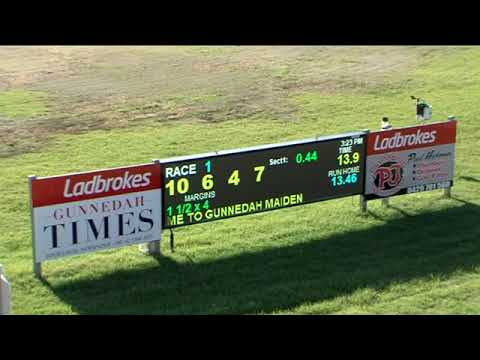In this sunny outdoor setting, an expansive grassy field is punctuated by a prominent digital scoreboard positioned centrally. This scoreboard, primarily black with illuminated yellow, green, and blue numerals and letters, provides details of a race, indicating "Race 1" at the top. Below this, the numbers "10, 6, 4, 7" are displayed prominently, followed by "Margins: 1.5 by 4". At the bottom of the scoreboard, it reads "M.E. to Gunnedah Maiden." The scoreboard is flanked by two signs with the Ladbrokes branding in red and white, each featuring additional text. On the left sign, it says "Gunningham Times," and on the right, partially legible, it includes "PJ." The scoreboard casts a large shadow on the grass, emphasizing the clear, bright conditions of the scene, and the background features patches of dirt with sparse grass coverage.